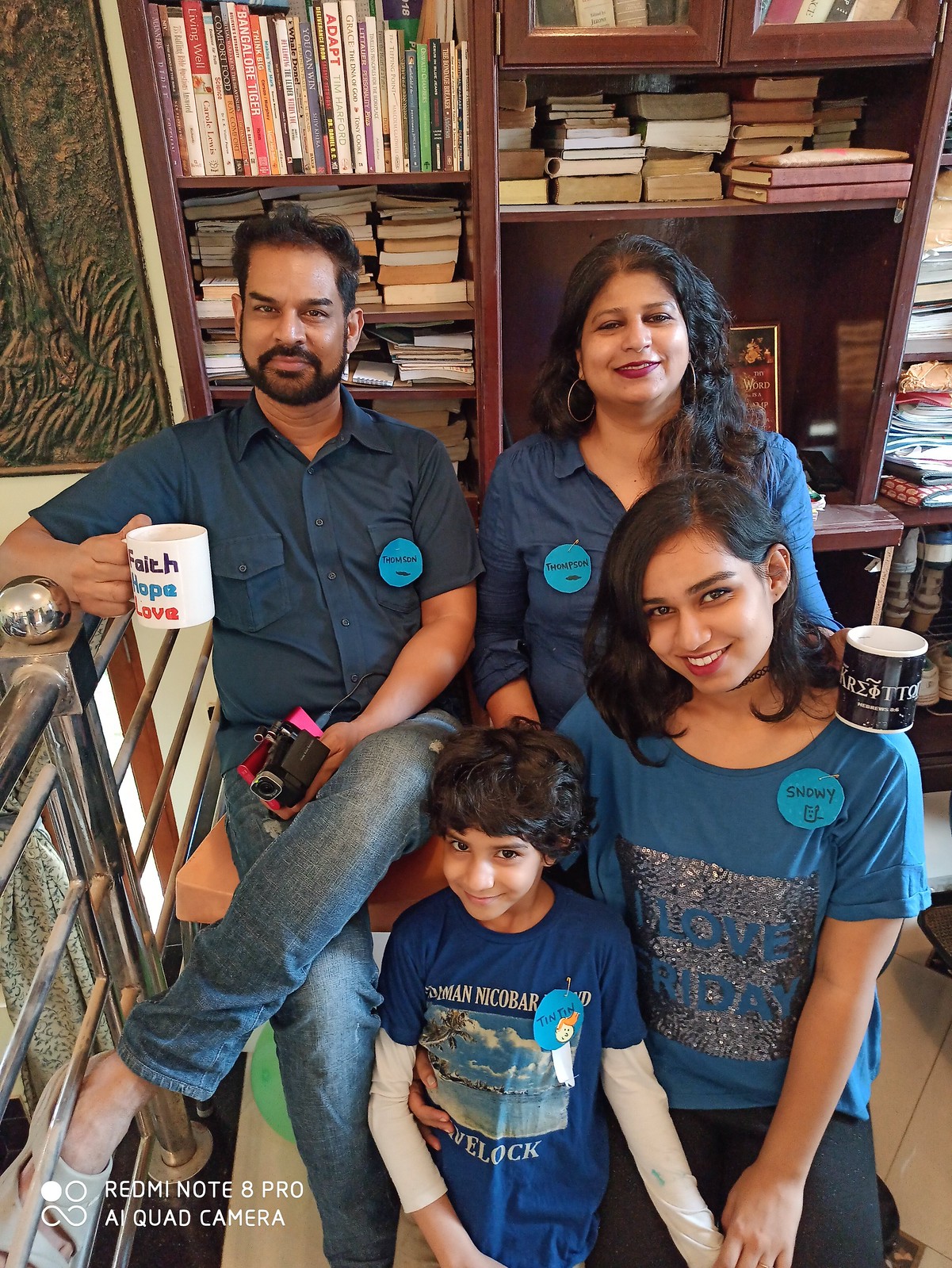In this detailed and charming photograph, a family of four is seen smiling and posing for the camera in what appears to be an office or business setting. The backdrop is a large bookcase filled with books, some stacked vertically while others are arranged horizontally, along with a few framed pictures and a wooden carving on the left side. Seated in the back row on a bench with a peach cushion are the mother and father. The father, on the left, has his right elbow resting on a countertop while holding a white mug inscribed with "faith, hope, love" in his right hand and a camera in his left. His left leg is casually crossed over his right. The mother, beside him, has long, dark, curly hair. She is holding a black coffee cup slightly above her daughter's shoulder with her left hand, while her right hand rests on her lap. 

In the front row, kneeling on the floor, are the two children. On the right is the older daughter, potentially a young teenager, wearing a blue T-shirt with graphics and a name tag that reads “Snowy.” Beside her, on the left, is the younger son, who appears to be around five years old, also in a graphic blue T-shirt. Both children share their parents' eye-catching blue attire as the parents both wear matching blue button-up shirts. Each family member dons a round, light blue name tag, harmonizing their coordinated look.